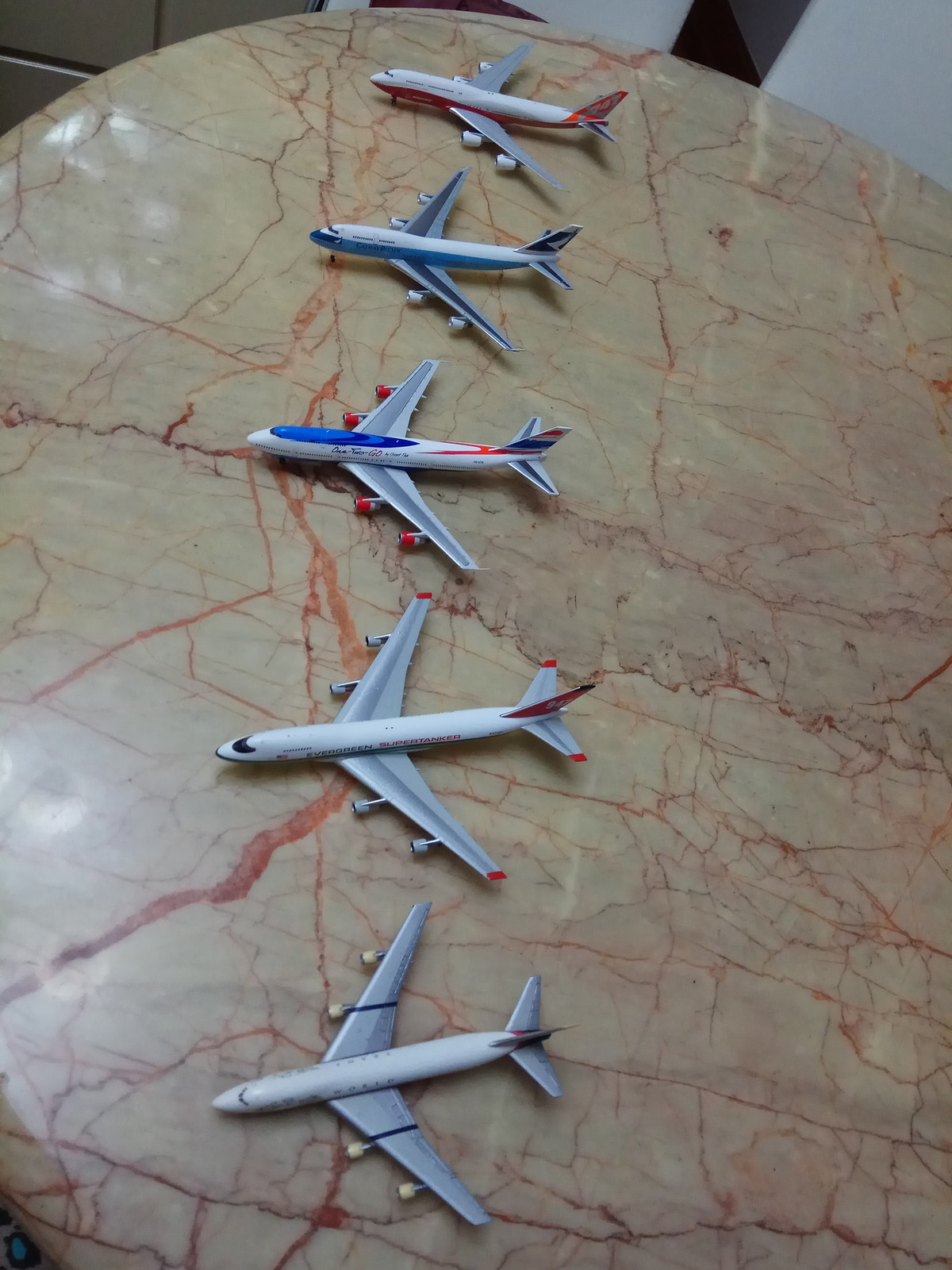The photograph captures a round, white marble table with distinctive reddish-brown veining, possibly appearing orange or beige depending on the perspective. The image is shot from above, clearly displaying five model aircraft aligned vertically from top to bottom along the table’s center. Each aircraft, appearing in shades of white or gray, features unique color accents distinguishing them from one another. The topmost aircraft sports red pinstriping along its side and a red tail. The second aircraft under it features blue pinstriping along both the side, wings, and tail. The central aircraft is adorned with a blue top, gray wings, and a yellow stripe extending towards a red and blue tail. The fourth aircraft has subtle red hints, mostly concentrated on the tail sections. The fifth and final aircraft, primarily gray, is marked with two red hints on the tail section as well. The marble’s intricate, reddish-brown veining becomes more pronounced near the left side of the image, creating a visually compelling contrast with the model aircraft. The corners of the photo show darker grey tiles on the upper left and a lighter grey with what appears to be a brown or black bar in the top right, adding depth and context to the setting.